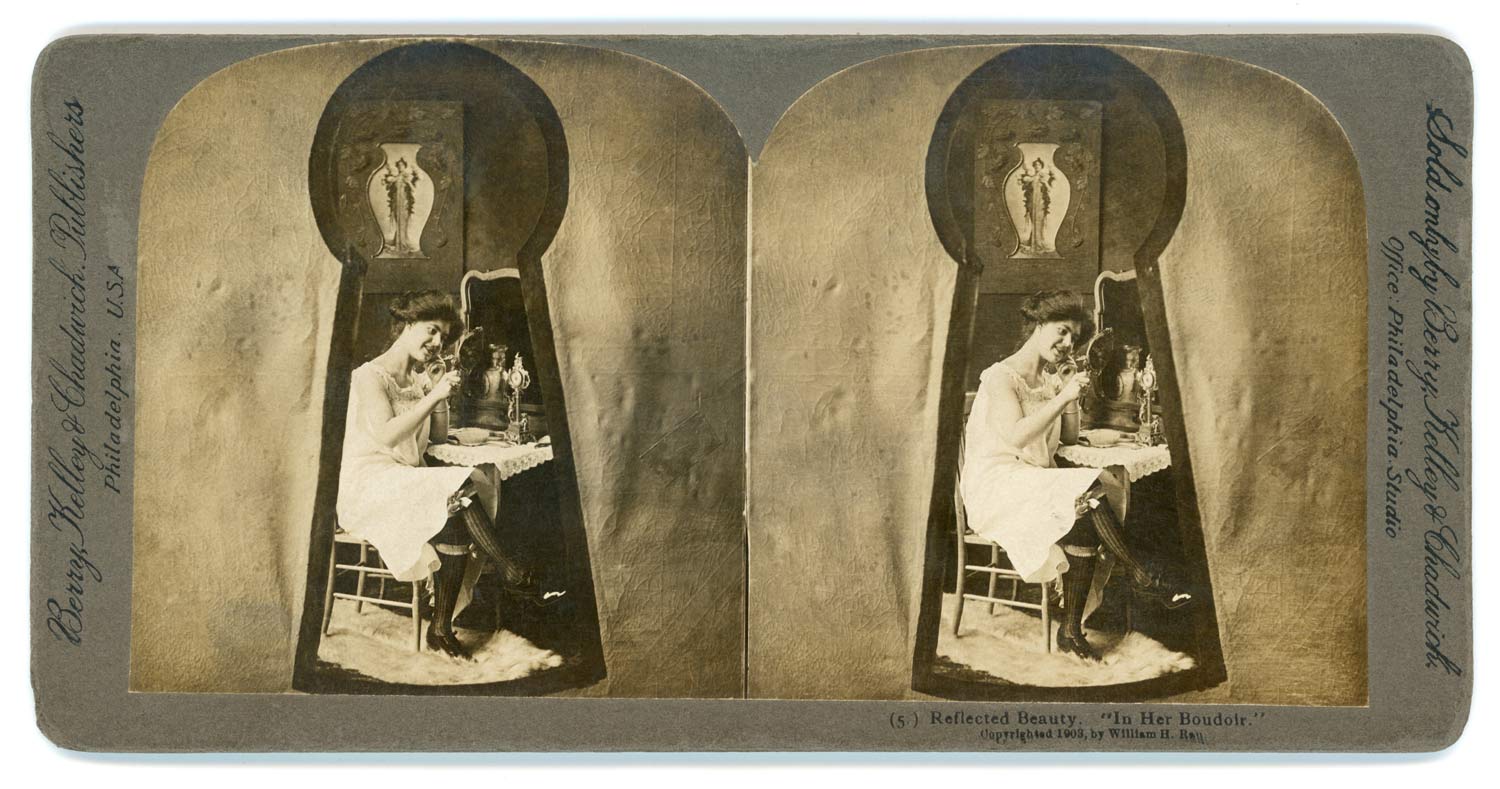The image is divided into two side-by-side black and white panels, both featuring a similar or identical scene. Each panel provides the view through a keyhole, reminiscent of an old-fashioned, barrel-shaped keyhole with a rounded top and a broader base. The keyholes frame the image of a woman sitting at a vanity table, dressed in a long white gown or undergarment and long stockings. She is seated on a small chair with a white rug beneath her feet. 

The woman is holding a mirror in her right hand and appears to be applying makeup, while her left hand rests under her chin. In front of her on the table, which is covered with a small tablecloth, stands a larger mirror. Behind her, there is a picture of a woman standing, contributing to the intimate setting. Both panels present the same scene, suggesting an early 1900s photograph due to the style and clothing depicted.

The background is a grayish-white, paper-like texture. Vertical text is scripted along the left and right edges of the image. On the left side, it reads, "Berry, Kelly, and Chadwick Publishers, Philadelphia, USA," and on the right side, "Sold only by Berry, Kelly, and Chadwick Office, Philadelphia Studio." An additional caption below the right panel states, "Reflected Beauty in her Boudoir, copyright 1905 by William [last name]." The overall image gives a nostalgic glimpse into a private moment, seen through the voyeuristic perspective of a keyhole.